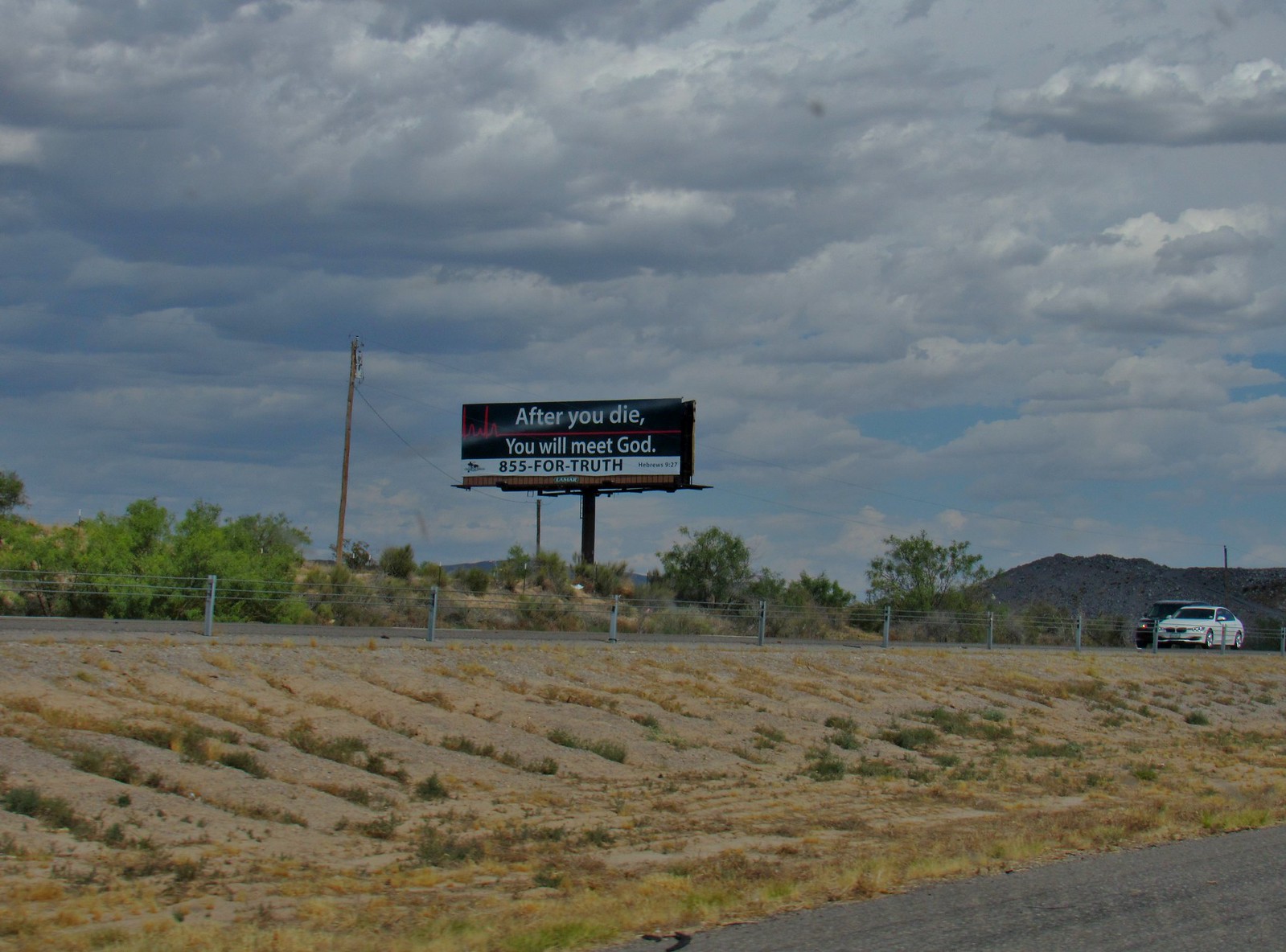This image captures a billboard set against a desolate, brown landscape with patches of green grass and yellowing plants. The photo is taken from an angled perspective, likely from a moving vehicle. In the bottom right corner, part of the roadway and a median dividing the oncoming and outgoing traffic are visible, populated with burnt grass and dirt. Two cars, a white one and a black SUV, drive along the road adjacent to a short, wiry fence with gray fence posts, which extends across the center of the photo lengthwise. 

The billboard, standing on a dark post, dominates the upper center of the image. It has a black background and features a red heartbeat line across the middle. The text on the billboard reads, "After you die, you will meet God," in white letters. Below this, a white banner with a phone number, "8554 Truth," is clearly visible. The sky is mostly cloudy, but enough light penetrates to suggest it is daytime, casting a subdued yet blueish hue in the background. In the far distance, hills or possibly low-lying mountains can be seen on both the left and right sides of the photo, adding a final touch of depth to the barren scene.